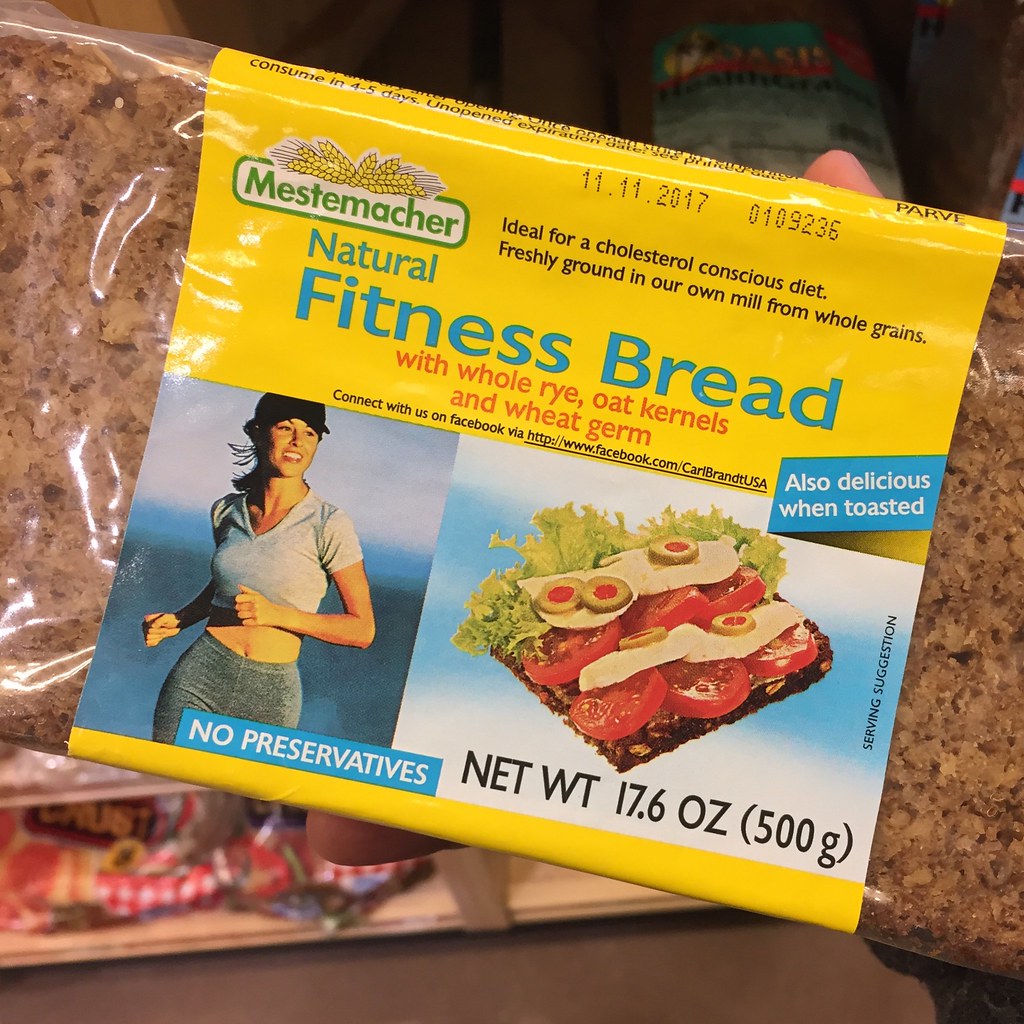The image captures a package of "Naturally Fitness Bread" with a predominantly yellow label and light blue lettering. The label highlights "Whole Rye, Oat Kernels, and Wheat Germ" in bold red letters. Below this, in small black lettering, it suggests connecting with the brand on Facebook via "http://www.facebook.com/CarlBrandtUSA". Additional information on the package includes the product being "Also Delicious When Toasted," "No Preservatives," and the weight of the package, "17.6 oz (500 grams)". The brand name, "Mestemacher," is featured in green letters, accompanied by a cartoon depiction of yellow wheat above it. The packaging proudly states that the bread is "Ideal for a Cholesterol-Conscious Diet" and emphasizes that the ingredients are "Freshly Ground in Our Own Mill from Whole Grains."